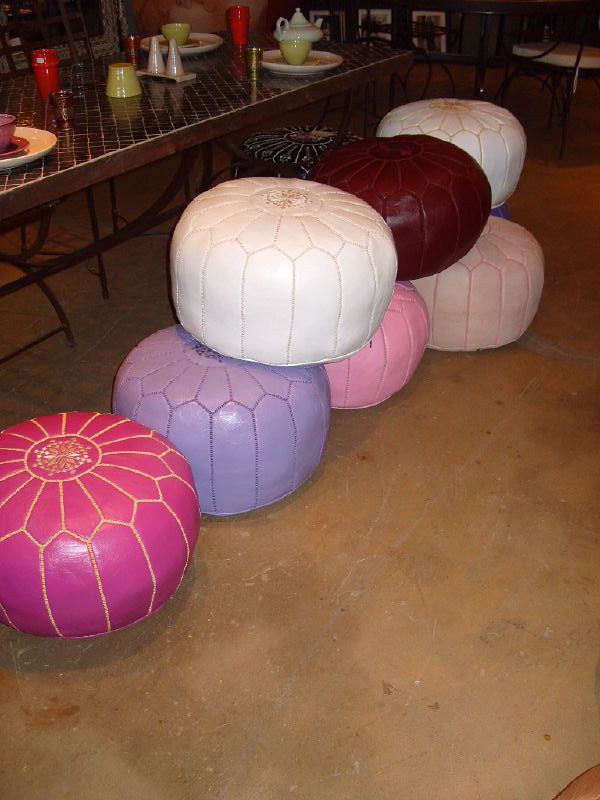This detailed image depicts a serene indoor setting, possibly within a Japanese-style teahouse. The focal point is a long, low table with a tiled or marble surface, suggesting a warm, earthy color palette that could range from brown to copper. The table is elegantly set for a meal service, featuring a variety of drink cups on saucers, some upside-down cups, and a centerpiece with salt and pepper shakers. A traditional teapot and what might be sake glasses add a cultural touch. 

Surrounding the table are nine seating poofs, arranged along the table with three neatly stacked on top of others, designed to resemble flower petals in shades like white, pink, maroon, lavender, and beige. These poofs, which are likely made from stitched panels of leather or a similar material, have a detailed flower pattern on top, featuring a central round piece surrounded by petal-shaped designs traced in complementary colors such as yellow on pink. The setup exudes a cozy and inviting atmosphere, perfect for a relaxed, communal dining experience.